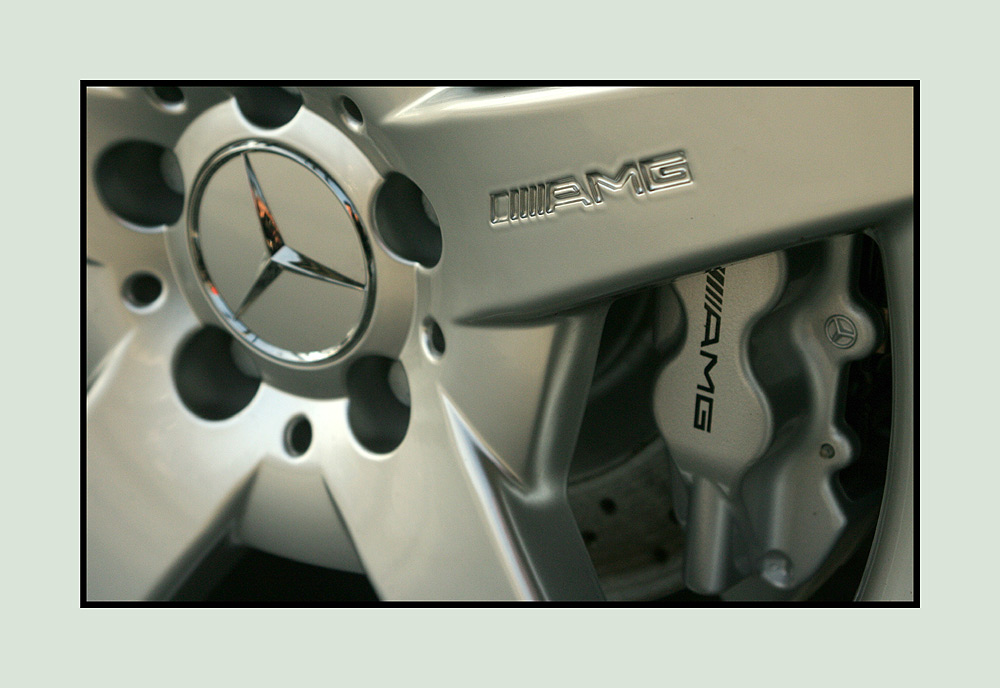The image depicts a detailed close-up photograph of a car's wheel, highlighting the tire, the metal rim, and the brake system. Central to the wheel, the chrome Mercedes-Benz logo, characterized by a three-pointed star enclosed in a silver circle, reflects its surroundings. The silver-painted hubcap, devoid of environmental reflections, prominently features the text “AMG” on both the metal rim and within the spoke structure. The overall color scheme is dominated by silver and gray tones, with reflective metallic accents enhancing the intricacy of the design.